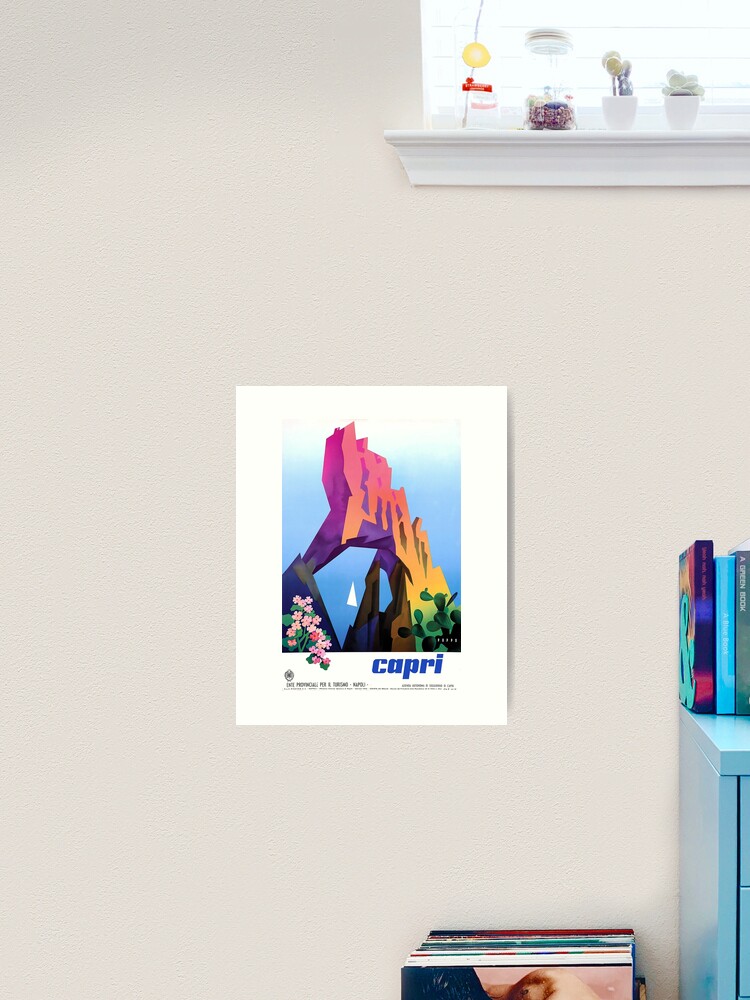The photograph depicts a minimalist interior showcasing a pale gray-lilac wall adorned with a vibrant, abstract art poster titled "Capri" in blue letters. The poster features a stylized, gradient-colored rock formation resembling a stone archway, with hues transitioning from pink at the top to yellow, orange, and green at the bottom. Surrounding the arch are green cacti on the bottom right and pink flowers on the bottom left. The wall also partially reveals additional elements: a light blue, minimalist dresser with three upright books, album covers slightly visible at the bottom, and a white windowsill with tiny potted succulents and jars containing miscellaneous items. The top edge of the photo captures a glimpse of the window, with sunlight spilling into the serene, modern-styled room.